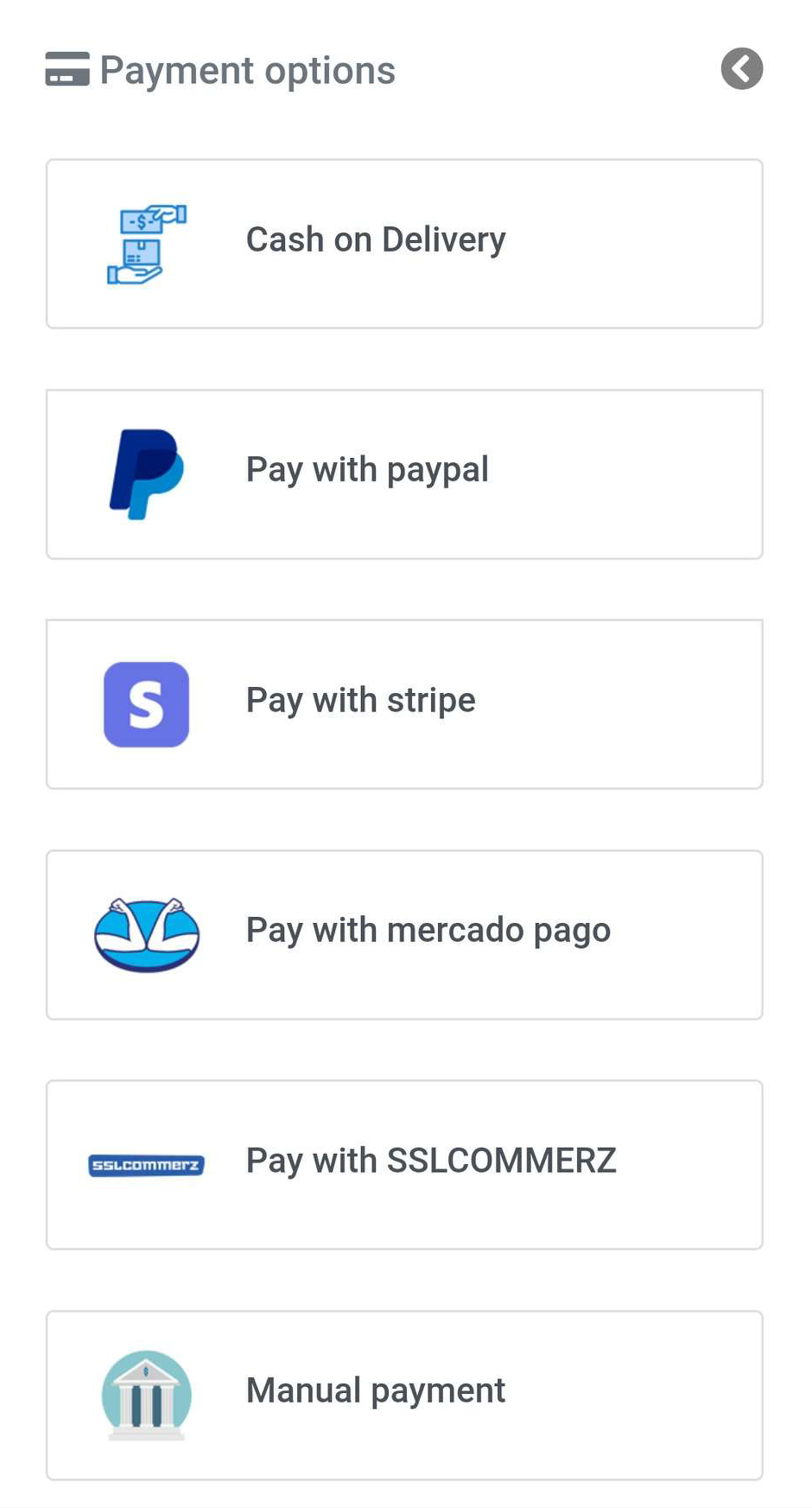This screenshot displays a list of various payment options available. At the top, in bold text, it reads "Payment Options". Below this header, there are six rectangular tabs outlined in faint gray. Each tab contains black text and an associated logo or icon.

1. **Cash on Delivery**: This option is represented by an icon of two hands, with one hand holding a bill featuring a dollar sign, and the other hand holding a box.
   
2. **Pay with PayPal**: The PayPal option is signified by a logo with two overlapping 'P's, one in dark blue and the other in light blue.

3. **Pay with Stripe**: This method is indicated by a blue square background with a white 'S' on it.

4. **Pay with Mercado Pago**: Depicted by an icon of an oval encircling the outline of two arms with fists raised and touching in a gesture of agreement or partnership.

5. **Pay with SSL COMMERZ**: This option's visual representation is missing from the description but it is included as the fifth tab.

6. **Manual Payment**: The last option listed is "Manual Payment", although the description does not specify its corresponding logo or icon.

Each of these options provides a distinct method for completing transactions, represented both by text and illustrative icons for easier recognition.